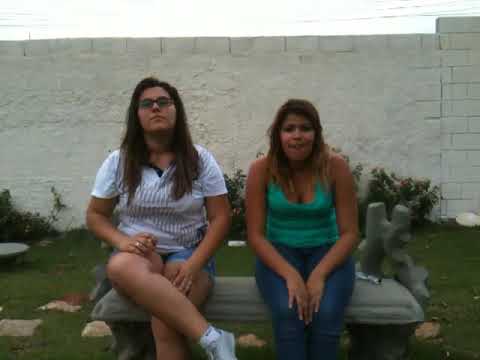In this image, two women are seated together on a gray stone bench in a grassy area adorned with various shrubs and stones on the ground, adding character to the scene. A white brick wall stands behind them with power lines visible against the sky above, suggesting an outdoor setting, possibly a park or residential yard. The woman on the left, who appears Caucasian with long brown hair and glasses, is dressed in a white, short-sleeved shirt with thin dark stripes and blue jean shorts. She has her legs crossed and is wearing white socks and white shoes. Notably, she sports a choker or necklace and a ring on her right hand. To her right, the second woman, who has a more tan complexion and might be of Hispanic or Central American descent, is wearing an aqua green blouse and dark blue pants. Her hair is also brown but shorter, and she sits with her hands clasped between her legs. The natural green backdrop of grass and bushes completes the serene outdoor environment.